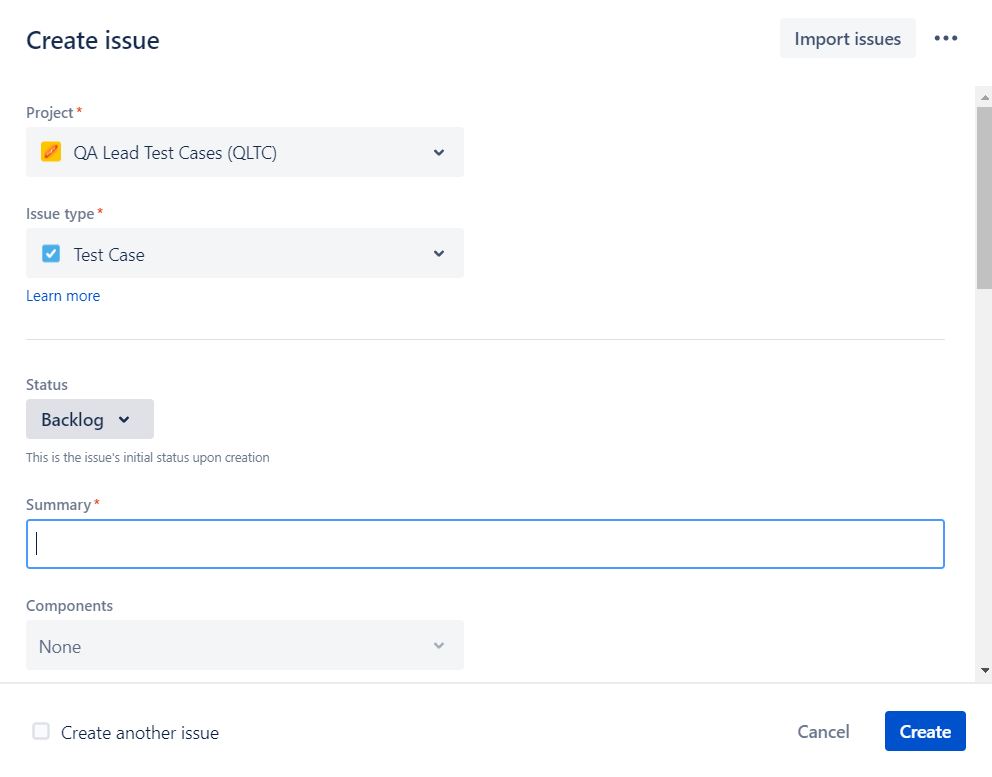The image depicts a user interface for creating an issue within a project management tool. The interface features a clean white background with a light gray button labeled "Import Issues" on the upper right side. Next to this button are three horizontal dots, indicating additional options.

On the left side, it reads "Project" in black text, accompanied by a red asterisk next to the "T" to indicate a required field. Below is a dropdown menu with the option "QA Lead Test Cases (QLTC)" selected.

The next section is labeled "Issue Type" with another red asterisk, denoting it as mandatory. Directly beneath is a pull-down menu displaying a blue checkbox with a white check mark labeled "Test Cases." There is a "Learn More" link in blue text beneath this section.

A thin gray line separates this from the next segment, which starts with "Status" and includes a pull-down menu set to "Backlog." Below this menu, instructional text states, "This is the issue's initial status upon creation."

Further down is the "Summary" field, marked again with a red asterisk. Adjacent is an empty data field with a white background and blue outline, indicating where the user can input the issue summary.

Below this is the "Components" section, with a drop-down menu currently showing "None." Another gray line follows, leading to the text "Create Other Issue" next to an unchecked gray box.

In the bottom right corner are two buttons: "Cancel" and "Create," the latter displayed in white font on a blue button. The interface prominently uses colors such as black, gray, white, red, blue, and yellow to differentiate various elements and statuses.